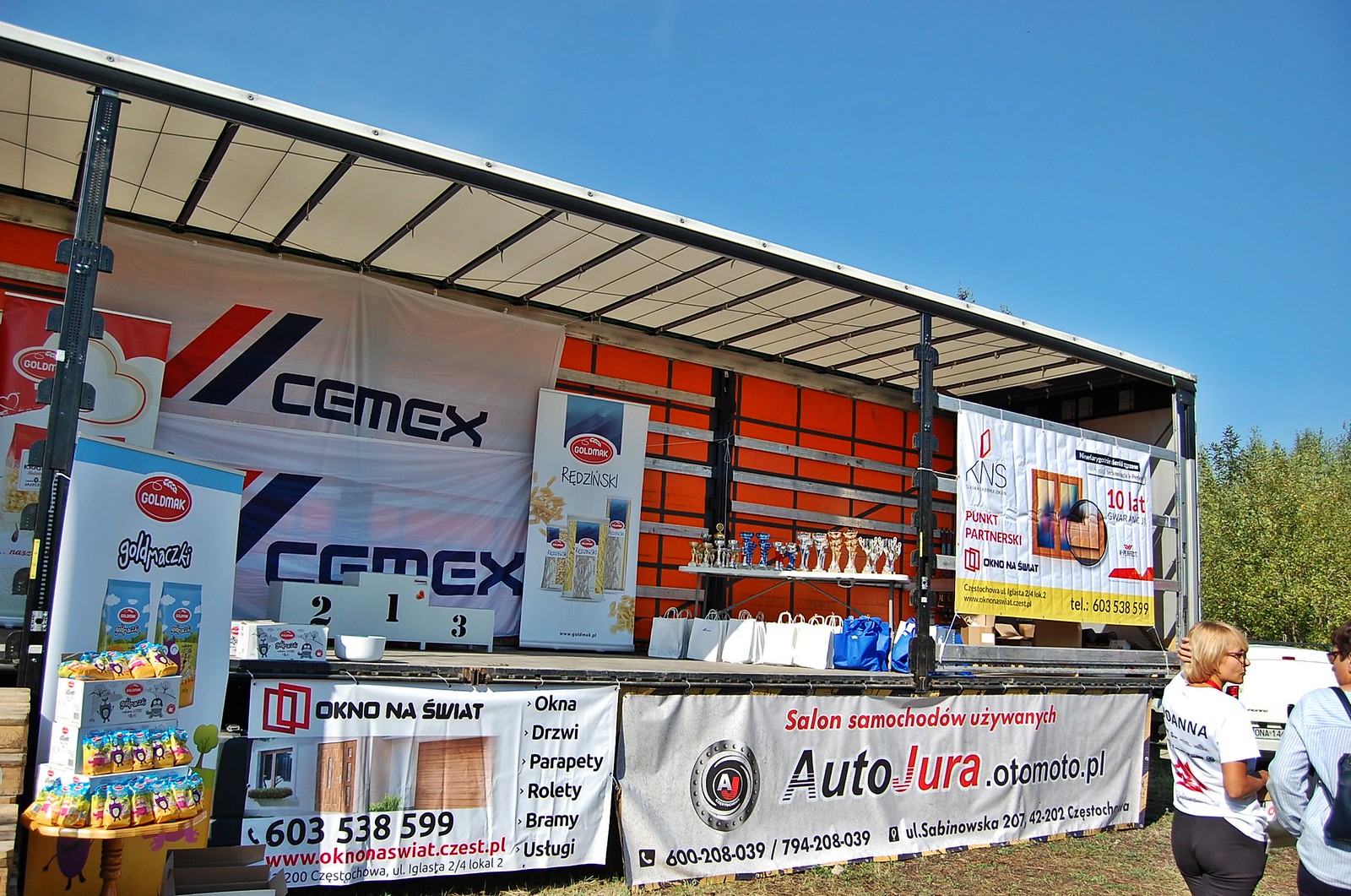This full-color photograph captures a vibrant outdoor scene on a sunny, cloudless day, with a vast expanse of blue sky. Centered in the image is a large display booth under a giant squared-off canopy, adorned with banners from various non-American sponsors, including Gold Racky's, Okno Naswiat Windows and Doors, and AutoJura.Otomoto.pl. The booth’s canopy and background feature a mix of orange, red, white, and blue, creating a lively and inviting atmosphere. 

Flanking the booth are green trees and a few people milling about, though the main focus is on the booth itself. Within the booth, you can see a stand designated for first, second, and third place winners, accompanied by gift bags and several trophies. There are rows of products that appear to include snack chips from a company named C-E-M-E-X, which also offers pretzels. Additionally, beautiful glass vases are displayed, with white and blue bags underneath, suggesting a wide variety of items for sale.

Among the visitors, a woman in a white shirt and a man in a blue shirt are clearly visible, both facing away from the camera, adding a human element to this bustling scene.